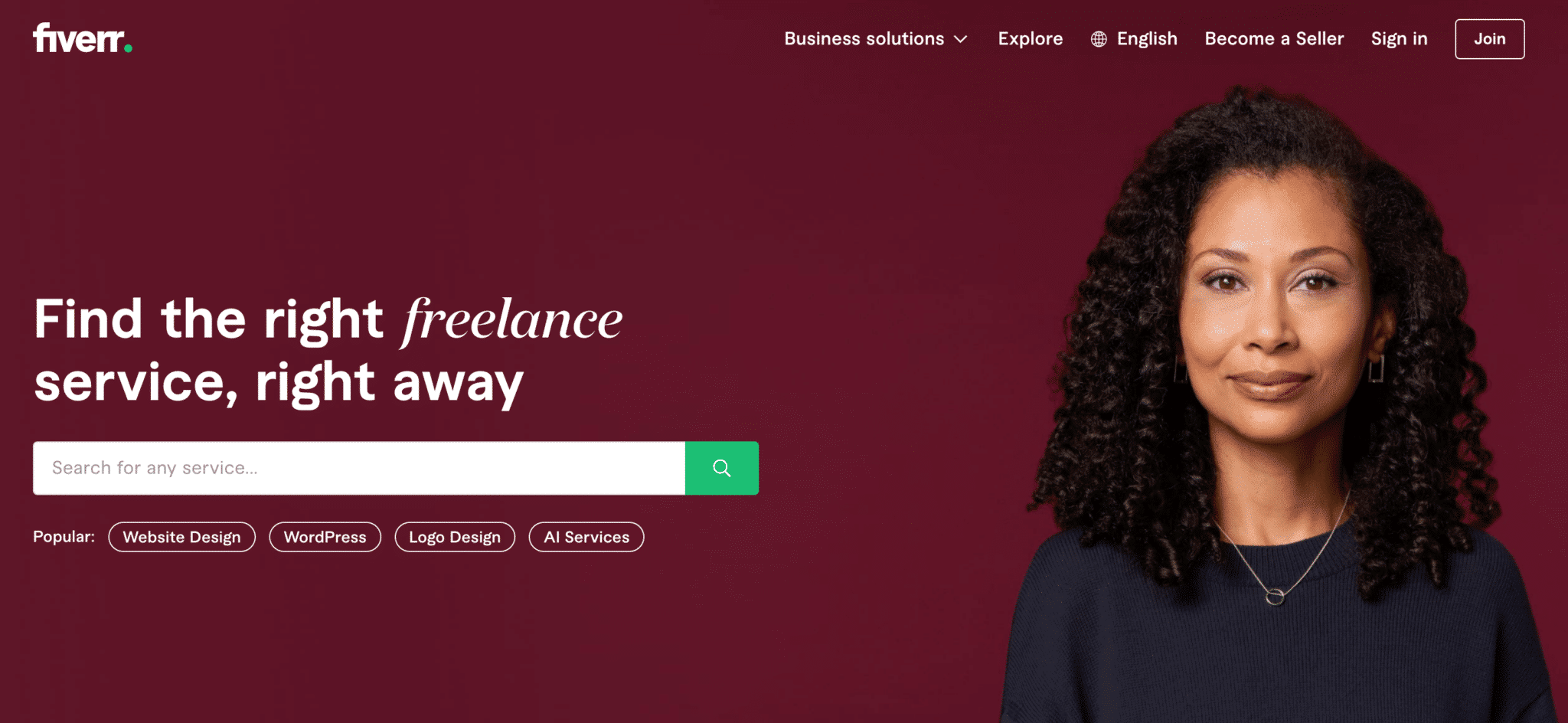Screenshot Description: Fiverr Homepage Interface

The image is a screenshot of the Fiverr homepage. Centered at the top left corner of the page is the Fiverr logo, written in lowercase with two 'r's at the end, followed by a small green dot. To the right of the logo, there is a horizontal menu bar featuring several options: "Business Solutions," "Explore," "English," "Become a Seller," "Sign In," and a prominent "Join" button.

The background of the page is a rich burgundy red. Occupying the left side of the screen is a welcome message in large, bold text that reads, "Find the right freelance service right away," with the word "freelance" italicized for emphasis. Directly beneath this text is a search bar accompanied by a green 'Search' button on its right side. Located below the search bar are four clickable tags labeled, "Web Design," "WordPress," "Logo Design," and "AI Services," providing quick access to popular freelance categories.

On the right side of the page is a stock photo of a woman in her 40s. She appears to be of African American descent, with shoulder-length curly hair and a slender face adorned with light makeup. She is also wearing a ring necklace, adding a touch of personality to her appearance.

The overall design elements and color scheme create an inviting atmosphere for users seeking freelance services.